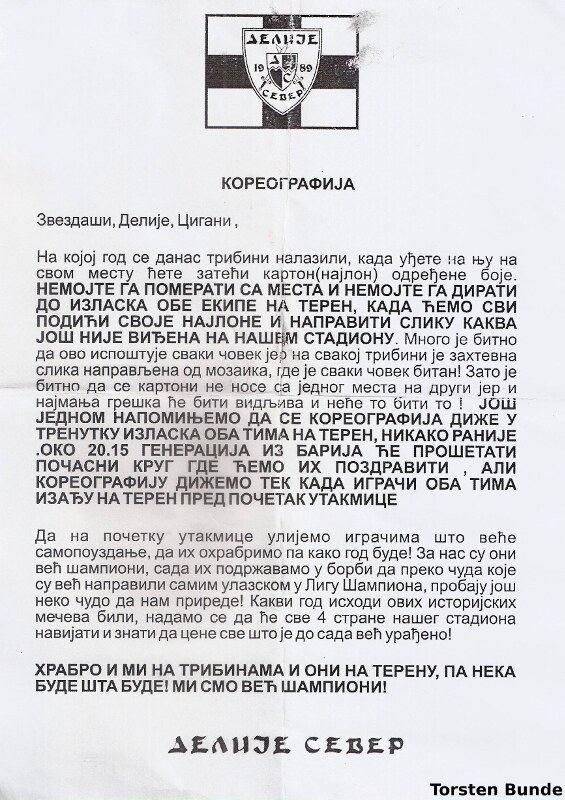The image is a photograph or scan of a printed piece of off-white or light gray paper featuring black text in Cyrillic script, making it illegible for those unfamiliar with the language. At the top of the page, there is an emblem that combines a flag and a coat of arms, reminiscent of the Swiss flag with its white field and dark cross. This emblem includes a heraldic shield containing various intricate designs, such as smaller shields within it, a sea, and potentially a hand, though details are difficult to make out due to the image's clarity and size. The shield also includes a date, which appears to be either 1980 or 1989. Some smudges are evident on the flag and within the body of the text, likely from smeared ink.